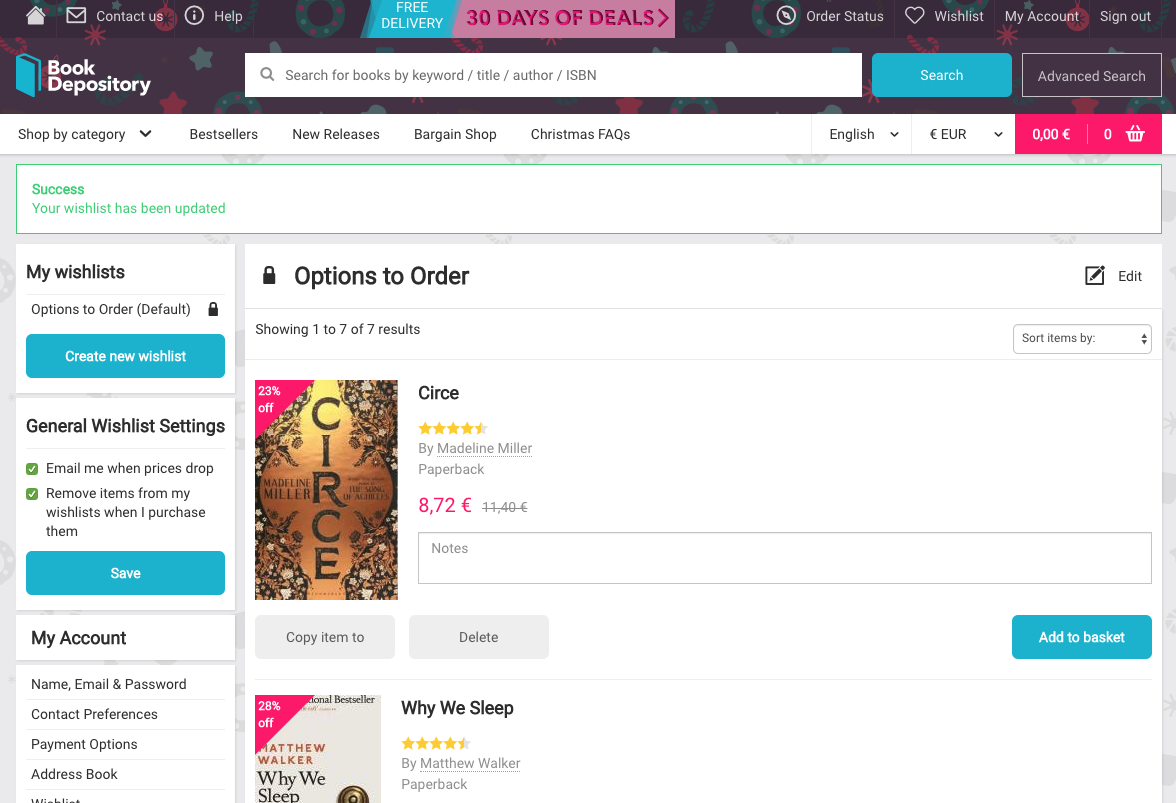The image depicts a webpage from the Book Depository website, clearly illustrating several key features and navigation options. At the top of the page, there's a prominent search bar, alongside a "Contact Us" button represented by an envelope icon. Adjacent to it are a Home button, a circled 'I' icon for Help, and a note indicating "Free Delivery" and "30 Days of Deals" highlighted in teal and pink.

Further down, the page offers various clickable options such as "Order Status," the ability to "Heart" items, add to "Wishlist," access "My Account," and "Sign Out." The navigation bar includes sections for "Shop by Category," "Best Sellers," "New Releases," "Bargain Shop," and "Christmas FAQs." The language is set to English, with currency options showing Euros and prices in pounds.

In the middle of the page, there’s a notification stating, "Success. Your Wishlist has been updated." The left side of the page features options to manage wishlists, including creating a new wishlist, accessing General Wishlist Settings, and enabling preferences like "Email Me When Prices Drop," and "Remove Items from My Wishlist When I Purchase Them." Below this, there are options to reorder, and it shows that two books are currently in the wishlist.